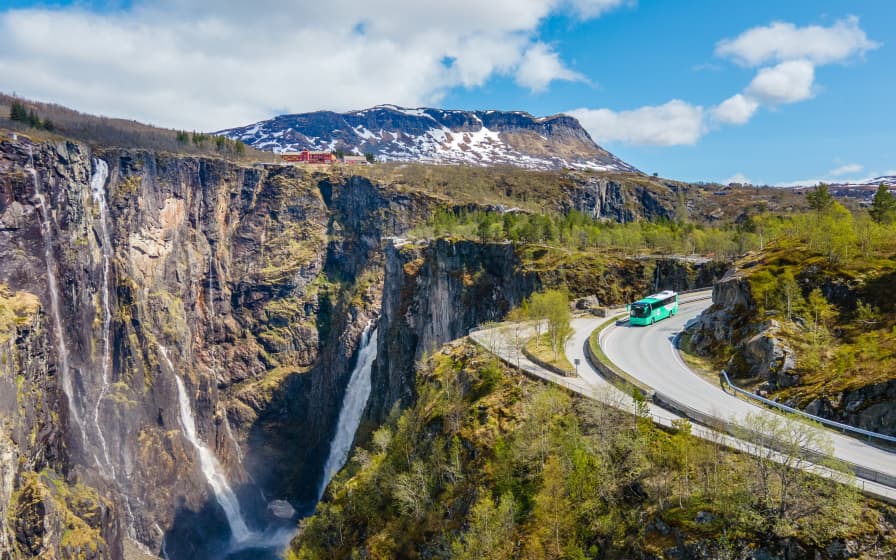The image captures a tour bus navigating a winding mountain road adjacent to a deep canyon with cascading waterfalls and a river at its base. The canyon features sheer cliffs made of stone and rock, while the road itself is paved and bordered by greenery. The green and white bus is traveling towards the right side of the photo, positioned centrally. In the far background, a vast mountain range colored in shades of brown and gray, with patches of snow, dominates the upper portion of the image. The sky above is clear with white, puffy clouds. Additionally, two buildings with metal roofs can be seen in the distance, one red and the other tan. No people are visible around or inside the bus, and the bus’s windows are dark and reflective. The entire scene is bathed in daylight, highlighting the lush green foliage that surrounds the road and canyon.